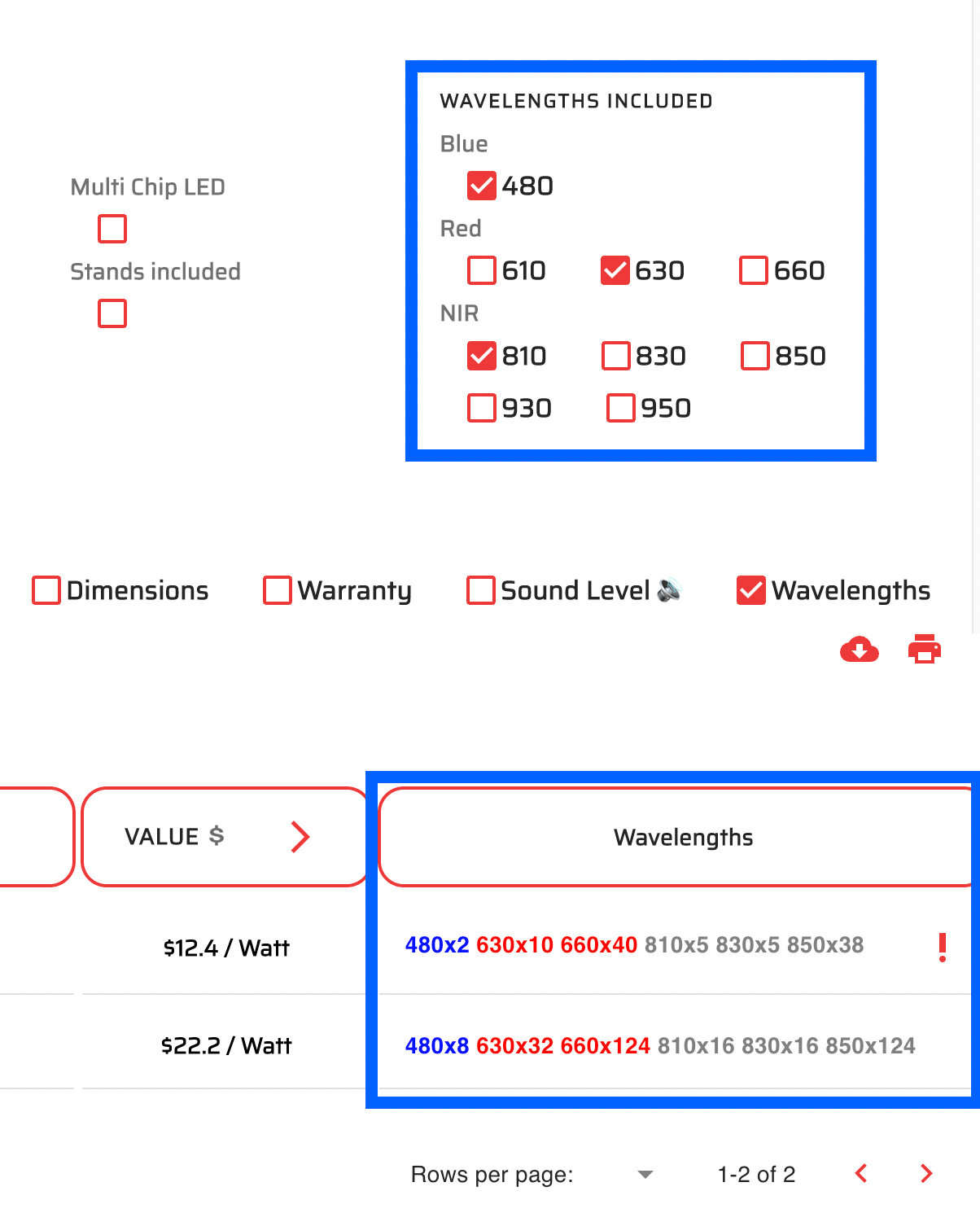A white page contains various technical details organized in a structured layout. On the left side of the page, starting from the top, a diagram of a multi-chip LED is displayed. Below this, there is a red box indicating certain specifications, although none of the options within the box are checked.

Encasing the entire content is a blue outline. Within this outline, there is a section labeled "Wavelengths Included," which lists several wavelengths such as:

- Blue (480nm) - checked
- Red (610nm)
- Red (630nm) - checked
- Red (660nm)
- NIR (810nm) - checked
- NIR (830nm)
- NIR (850nm)
- NIR (930nm)
- NIR (950nm)

Below this section, there are additional labels for "Dimensions," "Warranty," "Sound Level," and a checked "Wavelength." 

Adjacent to these labels, there are icons for "Download to Cloud" and "Print." Further down, there is a button labeled “Values” which features a red outline and a red arrow pointing to the right, with the word "Values" written in black inside the button. 

Beneath the "Values" button, two rows of data are presented. On the right side, there is another blue-outlined section labeled "Wavelengths," which contains additional details:

- The first row reads "12.4 W/Watt."
- Under the "Wavelengths" label, specific wavelengths are listed along with their quantities, including:
  - 480nm x 2
  - 680nm x 10
  - 660nm x 40

The page is detailed and structured to provide comprehensive information on the LED’s wavelength specifications and related technical data.